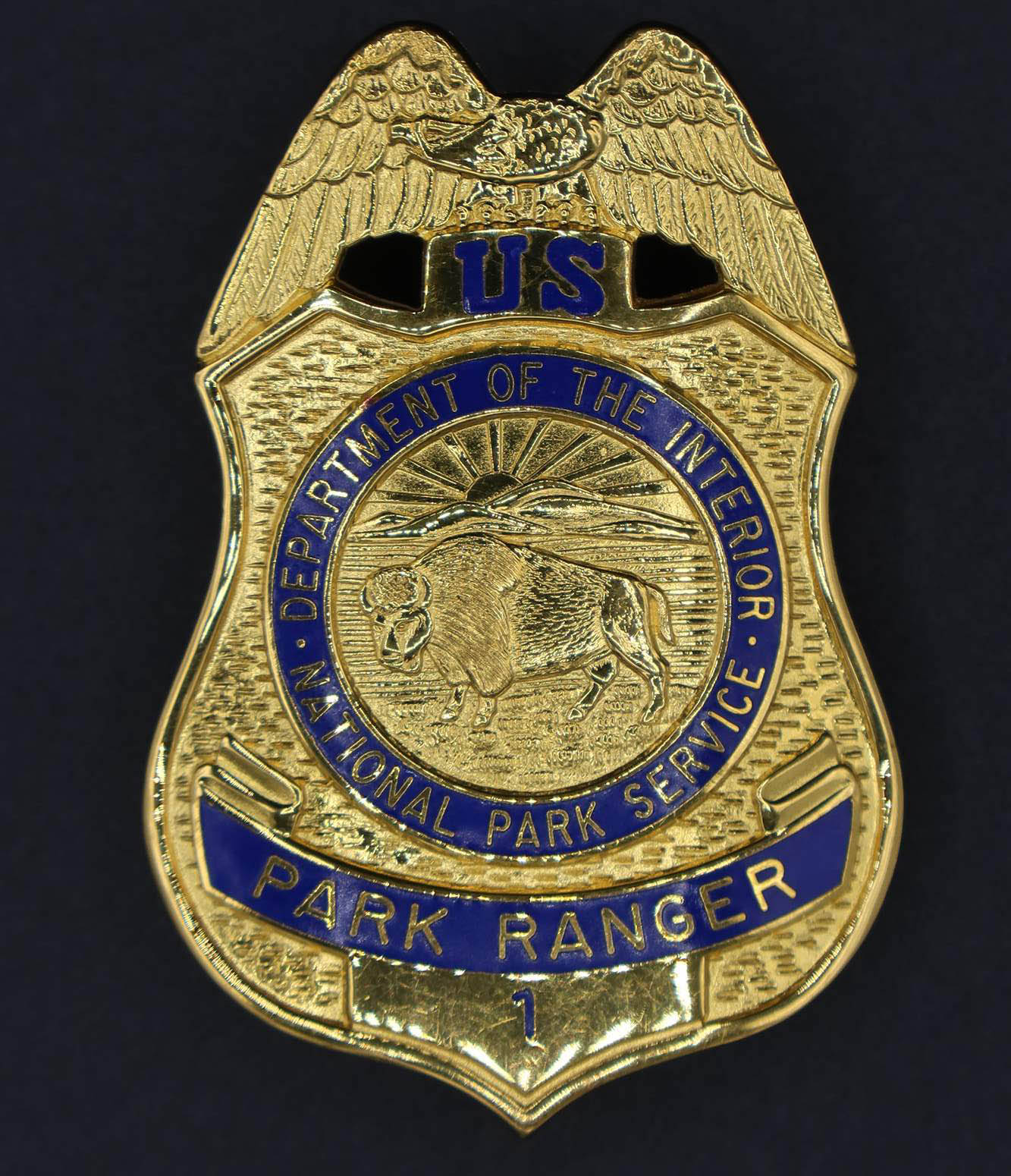This is a close-up photograph of a gold-plated park ranger badge set against a dark navy blue background. At the very top of the badge, an eagle with outstretched wings looks to the left, its talons resting on a small rectangular area that features the letters "US" in blue. The badge itself is shield-shaped with gracefully curved sides. Encircling the center of the badge is a blue ring with gold text that reads, "Department of the Interior, National Park Service." Within this circular frame, a buffalo etched into the gold face leftward, with a detailed scene of a mountain and a rising sun behind it. Toward the bottom of the badge, a scalloped blue banner proudly states "Park Ranger" in gold lettering, and directly beneath this banner is the number "1" inscribed in blue.